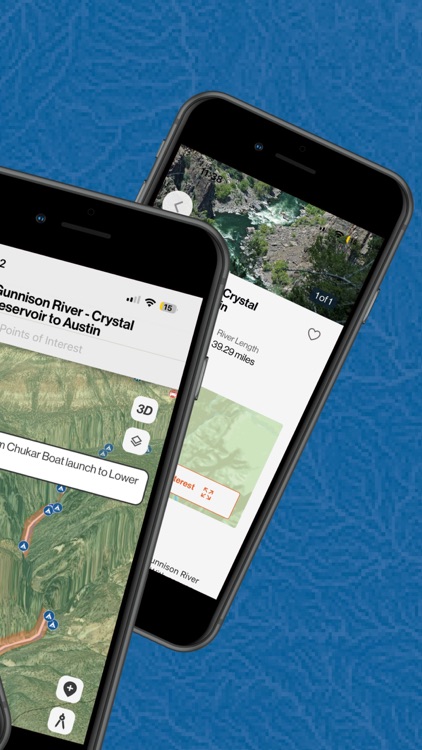This portrait-mode advertisement features an abstract blue background, interwoven with light blue veins that create a rough pattern. Dominating the foreground are two prominently displayed cell phones, both leaning towards the right. The first phone sits more centrally and slightly in the background, showcasing a black stripe across its top edge. Its screen displays a picturesque image of a river coursing between rocks, annotated with the text "11:38," an arrow pointing back, and "1 of 1". 

Beneath this, a large white section with bold text reads "Crystal," accompanied by a heart icon for favoriting in the upper right corner. Further details on the screen mention "River length: 39.29 miles." Below, there's a section with a green background containing the word "Interest," followed by a potential identification of the "Gunnison River."

The second cell phone is positioned from the left-center to the left-bottom of the ad, also leaning towards the right. The top stripe of this phone is white, displaying a "2" in the upper left-hand corner and "15" for 15% battery charge in the upper right. The screen displays text in bold: "Gunnison River - Crystal Reservoir to Austin." The background is gray with gray writing, making it somewhat difficult to read points of interest. This screen also features a large, 3D green map with dark green accents, labeled "Chukra Boat Launch to Lower," dotted with numerous small blue triangles.